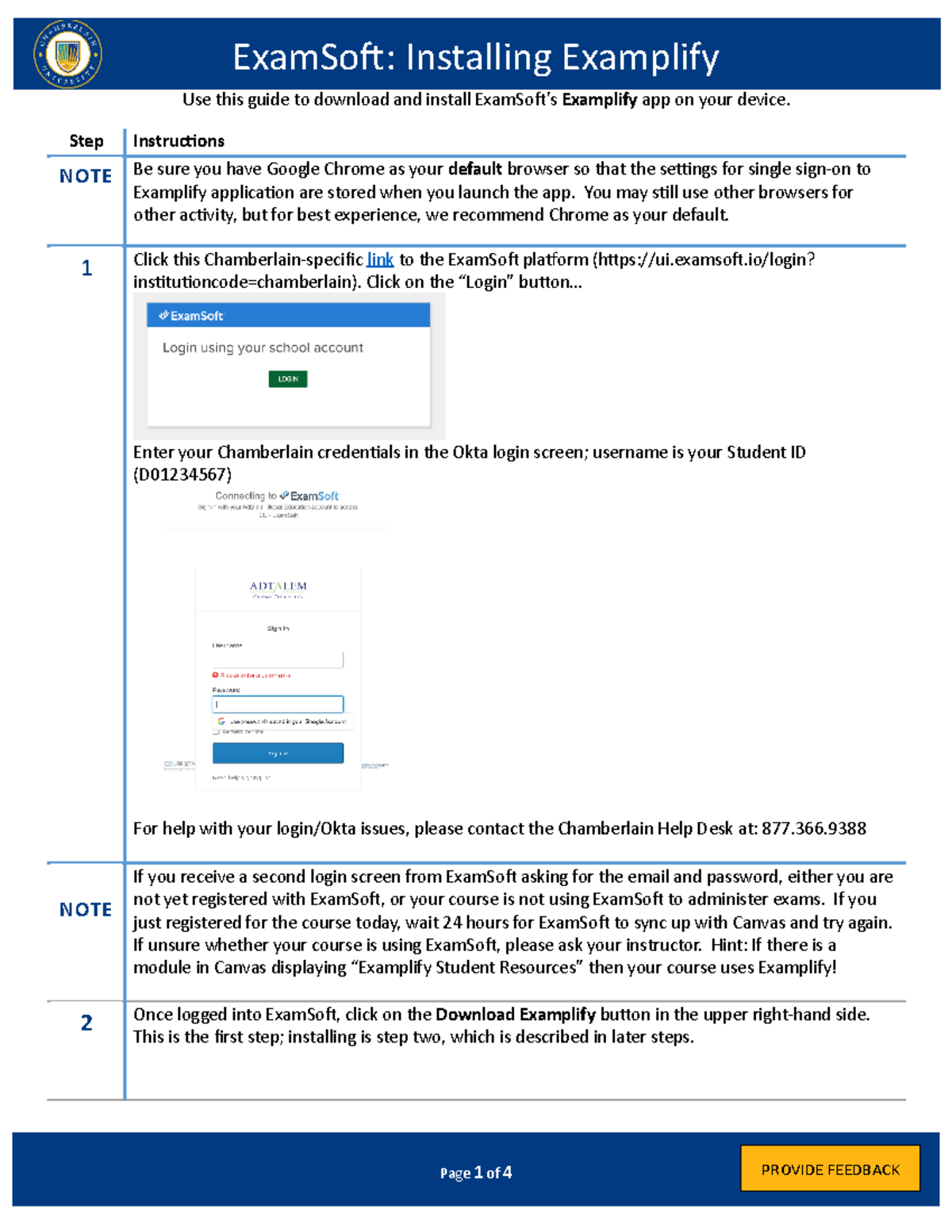Here is the cleaned-up and detailed caption:

The image features a blue border at the top with a circular emblem that reads "Chamberlain University" in white. Adjacent to the emblem, there is white text that says "Examsource.install.examplify". The background of the image transitions from white to black. Just below this, it states, "Use this guide to download and install the Examsource.Examplify app on your device."

The image is divided into two sections by a blue line that runs horizontally across. The left section is titled "Step," and the right section is labeled "Instructions." Below "Step," it says "Note" in blue, further divided by another blue line running horizontally. The opposite side of the line explains the note: "Be sure you have Google Chrome as your default browser so that the setting for the single sign-on exemplify application are stored when you launch the app. You may still use other browsers for other activities, but for best service, we recommend Chrome as your default."

Following the note, the left section lists "1," indicating the first step, which includes the instruction: "Click this Chamberlain-specific link and enter your Chamberlain credentials. The username is your student ID (formatted as D01234567)." A blue line continues vertically down the image and then horizontally across, breaking for another note labeled "2" in blue.

The note reads: "If you receive a second login screen for ExamSoft access and are prompted for your email and password, you either have not registered with ExamSoft or your course is not using ExamSoft to administer an exam." On the right, under "2," it states: "Once logged into ExamSoft, click on the 'Download Examplify' button located in the upper right-hand corner."

The image is visually structured to guide the viewer step-by-step through the process of downloading and installing the Examplify app, ensuring clarity and ease of understanding.